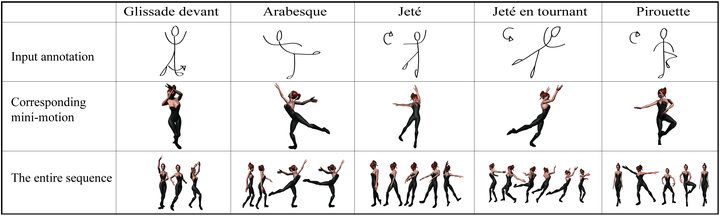The image presents a meticulously organized 5 by 3 table outlined with a thick black border, categorizing a sequence of ballet movements. The rows are labeled "Input Annotation," "Corresponding Mini-Motion," and "Entire Sequence." The columns are titled "Glissade," "Devante," "Arabesque," "Jete," and "Pirouette."

In the first row, simplistic stick figure illustrations show the various ballet poses, providing the foundational annotations for each movement. The second row features a rendered 3D cartoon-style female figure with black attire and red hair, accurately mimicking the poses illustrated above. The final row amalgamates these poses into full motion sequences, captured frame by frame. Here, the same cartoon woman is depicted multiple times within each cell, showcasing different stages of the movements: starting from three poses in the first sequence, then intensifying to four, five, and six poses in the following sequences, and concluding again with five poses in the final cell.

Overall, this image systematically visualizes the transition from simple line drawings to dynamic animations, illustrating the depth and grace of ballet movements.